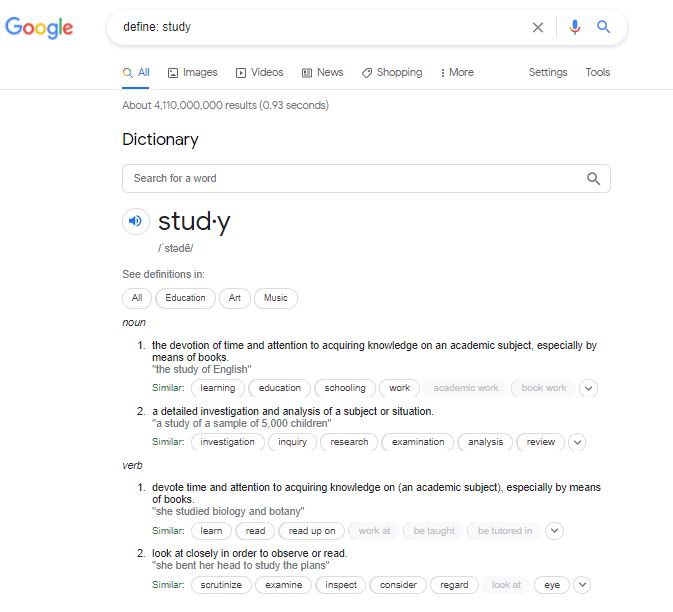A screenshot of a Google search results page is presented. On the left side, the iconic Google logo is visible, featuring its trademark blue, red, yellow, and green colors. Adjacent to the logo is a search bar displaying the query “define: study.” Below the search bar, various category options such as “All,” “Images,” “Videos,” “News,” “Shopping,” “More,” “Settings,” and “Tools” are listed. The “All” category is highlighted in blue, indicating it has been selected, while the rest are gray. The search results indicate approximately 4,110,000 results found in 0.93 seconds.

Below this, a dictionary section appears, with a search bar labeled "Search for word" and a text input showing the word “study.” The pronunciation of “study” is indicated as ‘stædē,’ and there is a blue button with a speaker icon that allows users to hear the word.

The definitions are organized under tabs labeled "All," "Education," and "Art & Music," each represented as buttons with a white background and gray outline. The noun "study" is defined in two primary ways:

1. “The devotion of time and attention to acquiring knowledge on an academic subject, especially by means of books,” exemplified by “the study of English.” Synonyms include learning, education, schooling, academic work, and bookwork.
2. “A detailed investigation and analysis of a subject or situation,” exemplified by “a study of a sample of 5,000 children,” with synonyms including investigation, inquiry, research, examination, analysis, and review. The example quote appears in gray.

This descriptive scene captures the essence of a Google search query related to the definition of the word "study," illustrative of the interface and features users interact with during their search.